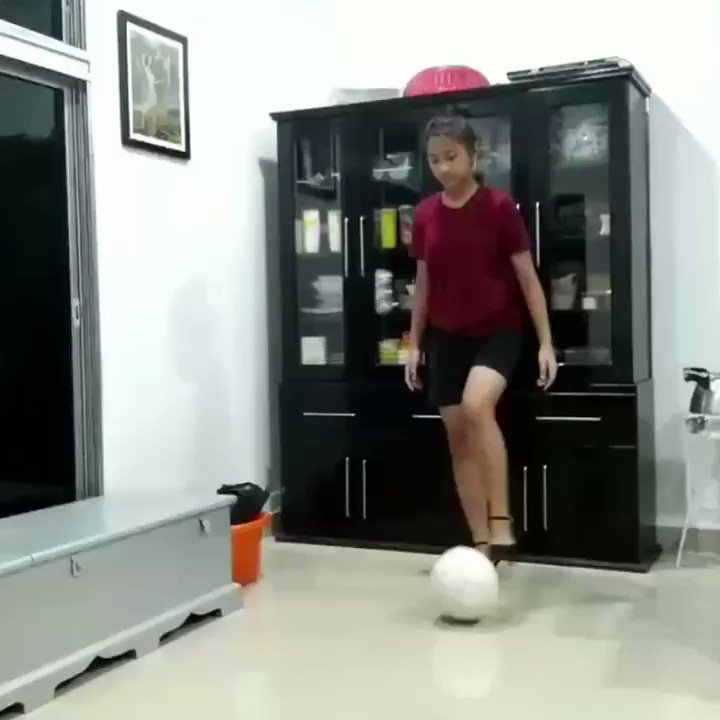In the image, a girl with black hair is captured in motion, as she prepares to kick a white ball on a gray floor. She is dressed in a burgundy short-sleeve crew neck top, black shorts, and black high-heeled shoes with straps. The setting appears to be indoors, with white walls and a gray chest positioned to her right, under a window with two dark-tinted panels separated by a white metal frame. Behind her stands a black cabinet with a glass-fronted upper section displaying dishes and a lower section with shorter black doors. To the left of the chest, there is a red or orange bucket. The girl stands in the center of the room, her right knee lifted and hands at her side, focused on the ball below her. The room is adorned with a black-framed photograph with a white mat, hanging on the white wall. Additionally, there's a pink object on top of the black cabinet, and a small bin next to it. The overall atmosphere suggests the picture was taken at night or that the windows are heavily tinted.